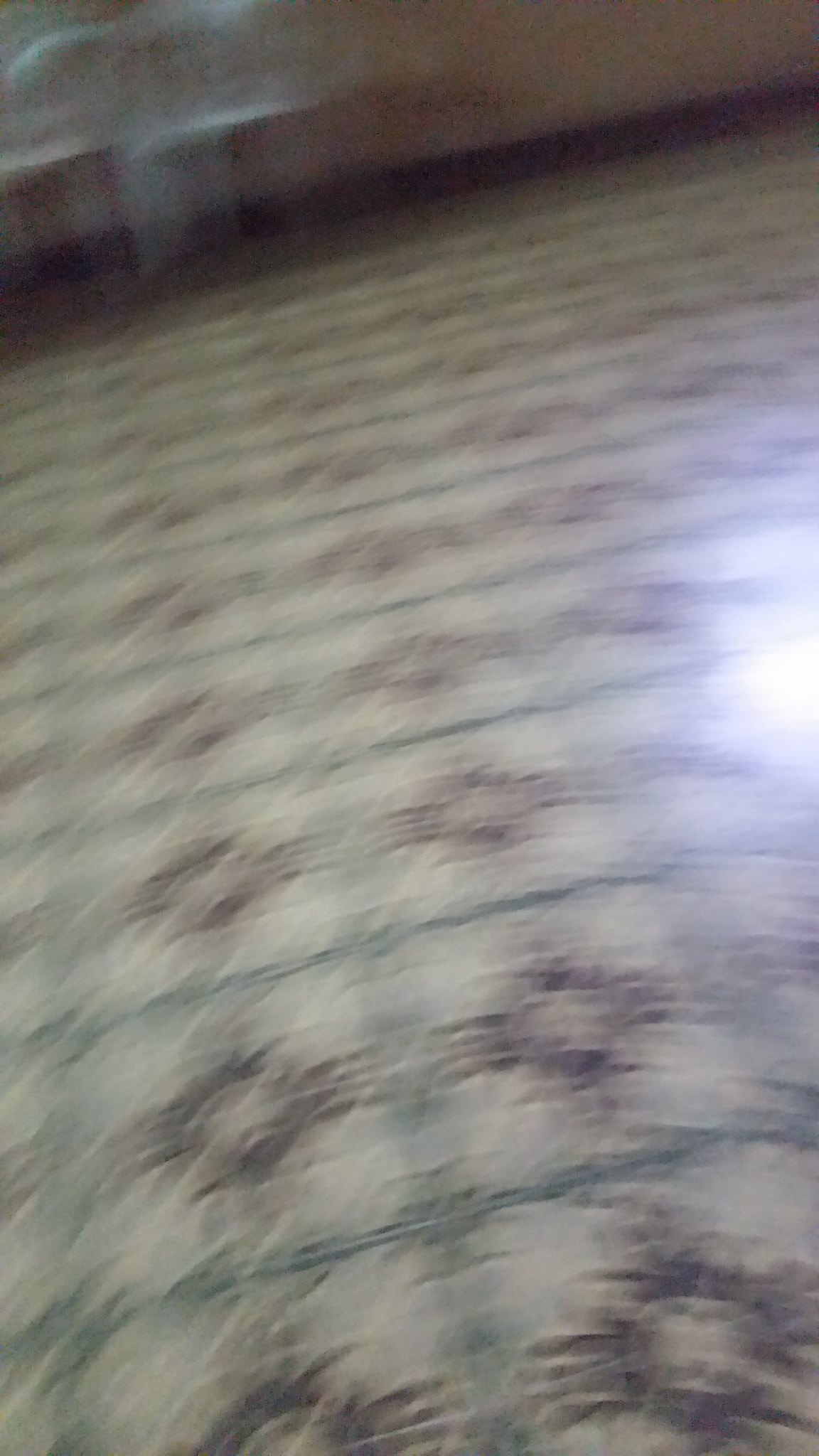This is an extremely blurry photograph capturing a detailed linoleum floor, viewed from a bottom-up angle. The image features a diagonally tilted perspective, with the left side lower than the right. The floor is composed of a series of white squares, each outlined in blue, and featuring a central red circle filled with yellow. Flanking the circle, three red stripes extend in both directions. An intricate and colorful pattern, blending red, brown, and possibly green designs, lies underneath the blur.

In the far background, where the floor meets the wall, there is a dark brown trim with a brown wall above it, suggesting a wooden or wood-paneled surface reminiscent of mid-20th century styles. On the left side, partially in view, are two white plastic chairs that appear ghostly due to the blurriness of the image.